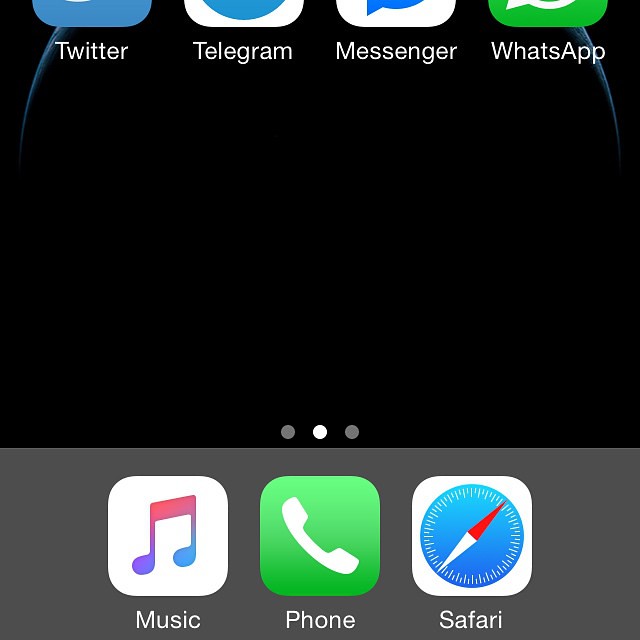A detailed view of an iPhone home screen displaying a variety of popular apps. Prominently featured are the Twitter, Telegram, Messenger, and WhatsApp apps, taking up half of the visible app area. At the screen's bottom, the Apple Music app, the standard Phone icon, and the Safari browser are neatly aligned in the dock. The screen background is simplistic, drawing attention to the app icons without additional clutter.